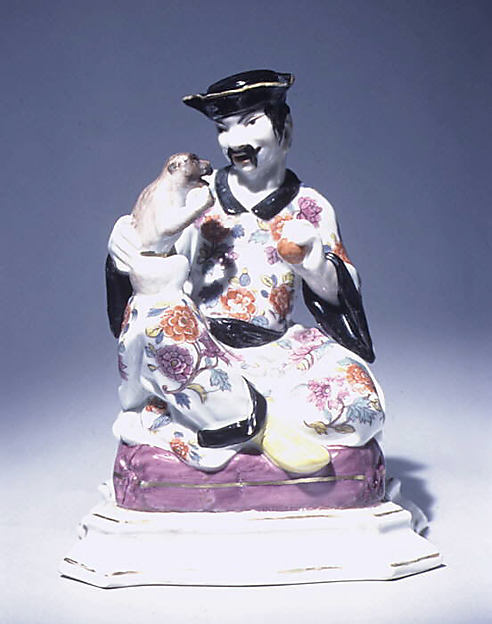The image showcases a detailed, small porcelain or ceramic figurine of an Asian man, likely representing a traditional figure, seated cross-legged on a purple base. The man wears an elaborate black hat with gold trim and has long black hair accompanied by a distinctive Fu Manchu-style mustache. His attire comprises a white robe with a black collar and belt, decorated with numerous colorful flowers, including orange blossoms, purple buds, and green leaves. The man is holding a piece of fruit in his left hand, which he is offering to a white and brown monkey positioned beside him. Both figures appear to be smiling, engaged in a peaceful interaction. This intricate figurine is set against a blue or light purple background and is mounted on a white base accented with gold lines.